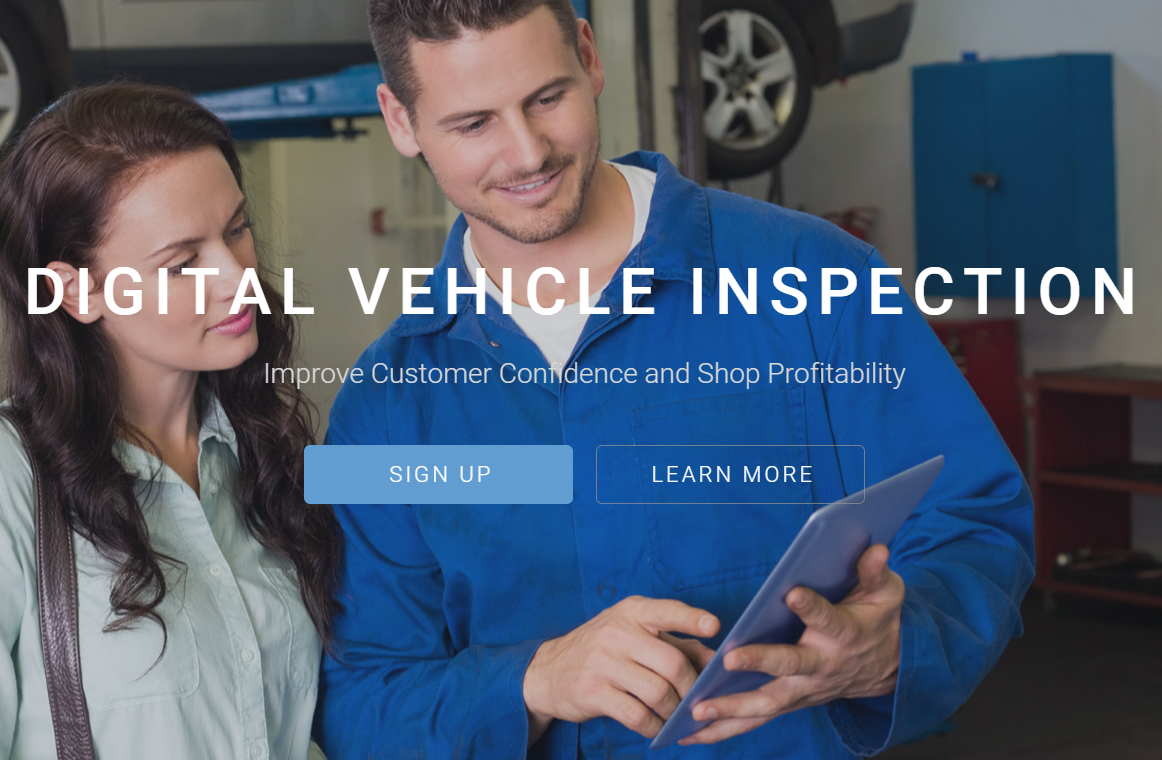In a vibrant and well-lit auto repair shop, a smiling Caucasian technician with short brown hair and a stubble beard holds a tablet, pointing at something on the screen. He is dressed in a blue jumpsuit with a white crew neck shirt underneath. Beside him stands a Caucasian woman with long, wavy dark hair cascading over her shoulders, wearing a light green button-up blouse and a brown purse strap over her right shoulder. She intently looks at the tablet, engaged in the discussion.

In the backdrop, a car is elevated on a lift, indicating the busy and professional environment of the workshop. Superimposed on the middle of the image in bold white capital letters are the words "DIGITAL VEHICLE INSPECTION." Beneath this, in smaller white letters, it reads "Improve customer confidence and shop profitability." At the bottom right of the image, a bright blue rectangle box prompts with the phrase "Sign Up," while a transparent box labeled "Learn More" in white type invites further action. The photograph is in landscape orientation and presents an engaging and professional atmosphere.